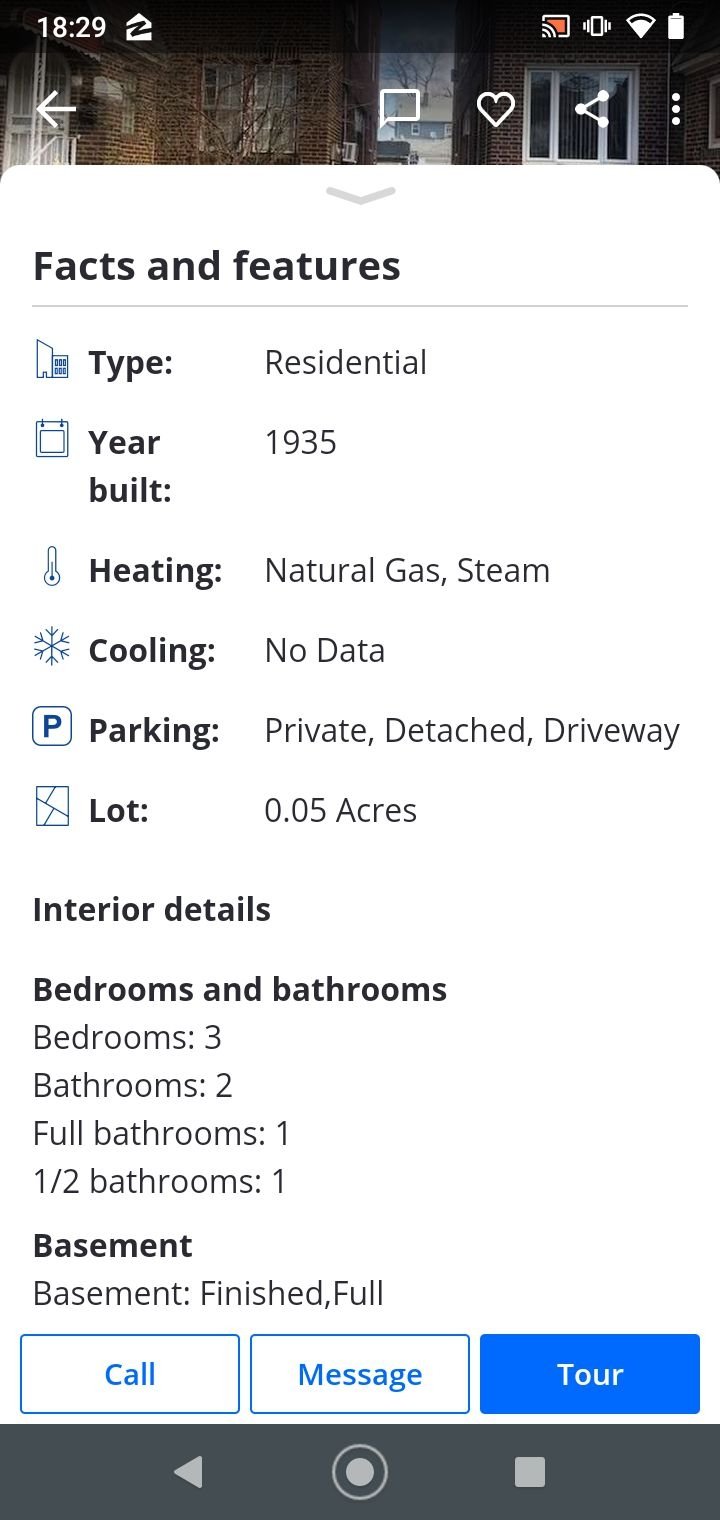Screenshot of a smartphone displaying a property listing on a real estate website, likely Zillow, in a military time format at 18:29 (6:29 PM). The phone shows full battery and a strong Wi-Fi connection. The top portion of the screen features a partially visible image of a house. Below the image, property details are visible: it is a residential home built in 1935, featuring three bedrooms and two bathrooms. The primary utility mentioned is natural gas, with little mention of acreage, highlighting the main features of the property.